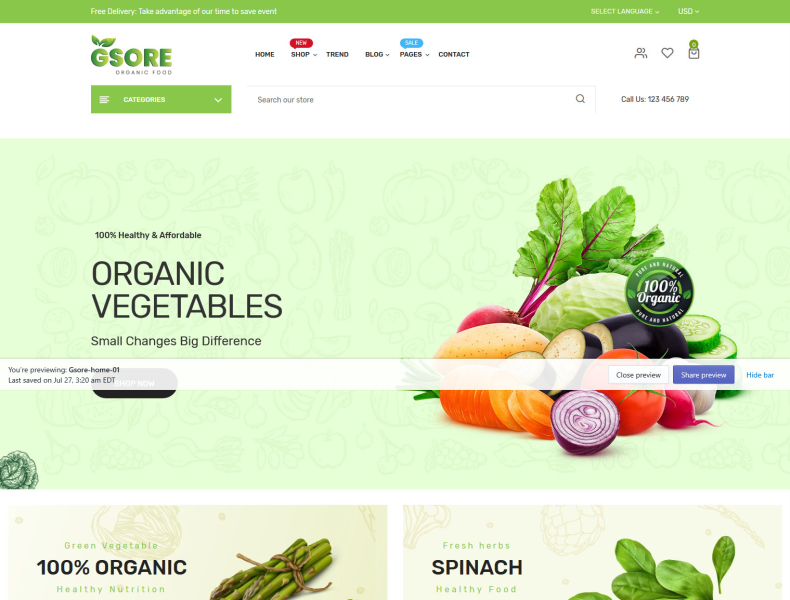This image is a screenshot from the G-SOR Organic Food website. Prominently displaying G-SOR's green logo, the website features a vibrant, lime green categories box. A large, captivating image of assorted vegetables dominates the front page, complemented by a green background adorned with vegetable stencils. Bold text declares, "Organic Vegetables - 100% Healthy and Affordable. Small Changes, Big Difference." The showcased vegetables include tomatoes, cucumbers, radishes, carrots, and sliced eggplant, all labeled as organic. Above this visual, a seal certifying "100% Organic" is visible.

Additionally, a translucent white stripe runs horizontally across the middle, indicating that the viewer is previewing "G-SOR Home 01," last saved on July 27th at 3:20 AM EDT, with "Close Preview" and "Share Preview" buttons displayed in purple.

Beneath the main section, there are two smaller sections: the left one highlights "100% Organic" asparagus, and the right one emphasizes "Fresh Herbs & Spinach" next to an image of spinach.

At the top of the page, there is a search bar, a customer support phone number (1-2-3-4-5-6-7-8-9), a language selection option, a shopping cart icon, and several navigation tabs for Home, Shop, Trend, Blog, Pages, and Contact.